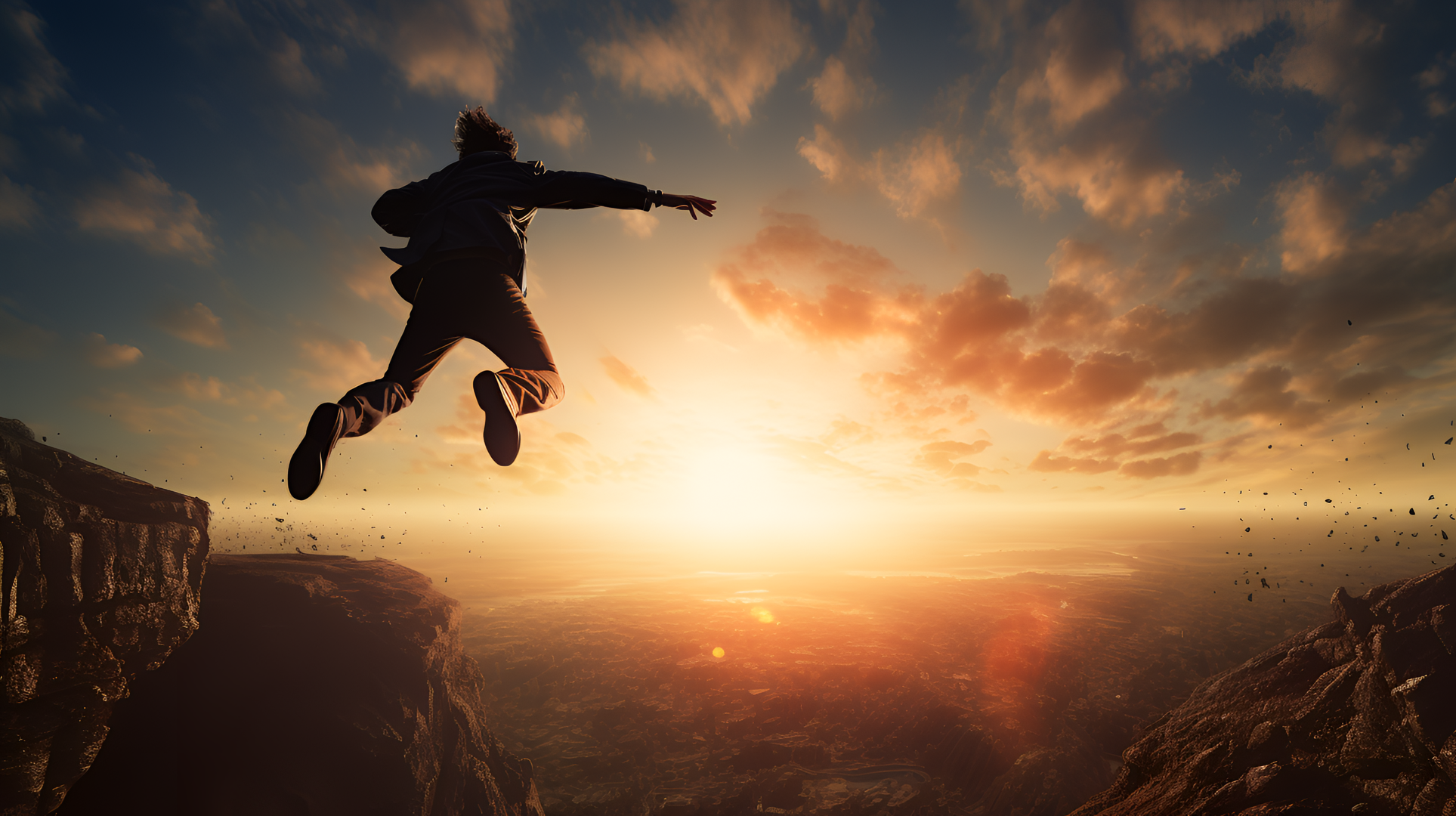The image captures a breathtaking scene of a person mid-air, likely base jumping, off a rugged cliff during a vivid sunset. The jumper, clad in a dark jacket, brown pants, and sneakers, has their arms and legs fully extended as they soar away from the rocky ledge. Their hair streams behind them, adding to the sense of motion. The sky above transitions from a deep blue to a vibrant mix of white and orange clouds, illuminated by the sun's golden rays that dominate the center of the scene. Below, the vast expanse of land stretches out, framed by jagged cliffs and scattered pebbles, giving a sense of height and grandeur to the leap.